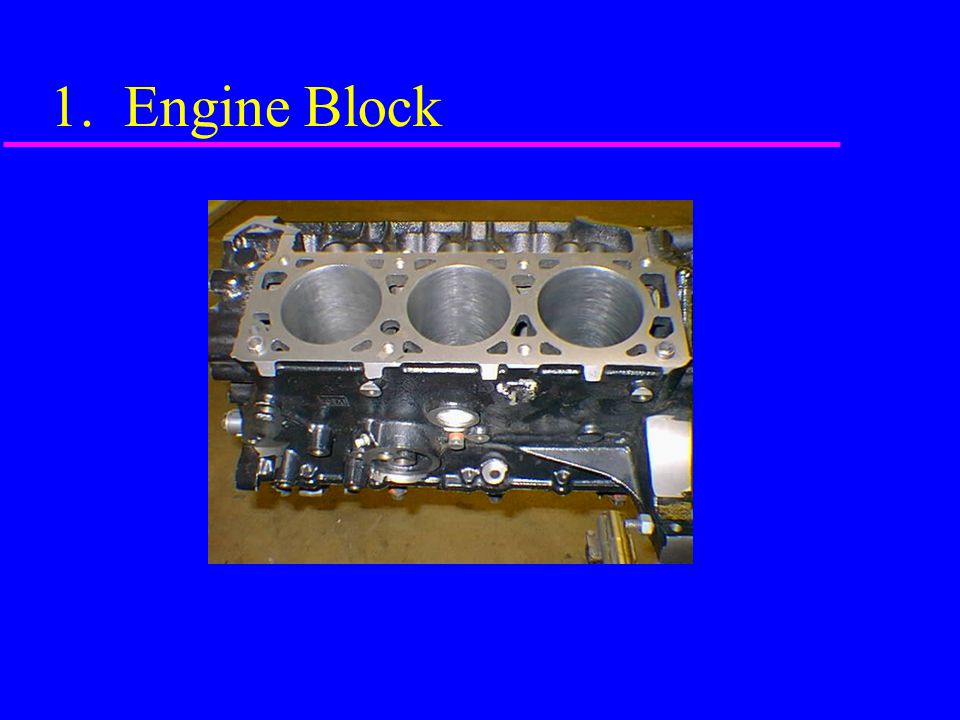The image features a bright blue background with the text "One Engine Block" at the top, written in Times New Roman font and displayed in a yellow color. Below the text is a pink dividing line, separating the label from the central subject: a silver metallic engine block. The engine block, part of a larger engine mechanism, is depicted as a flat rectangular panel with three large, circular cut-outs that penetrate the metal, creating visible holes. It rests on a dark brown surface, indicating a setting where engine maintenance or inspection occurs before the block is reinstalled for use.